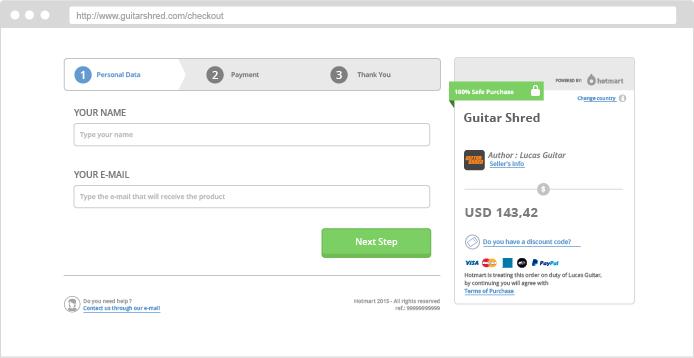**Caption: Detailed Overview of the GuitarShred Checkout Webpage**

At the top of the GuitarShred checkout webpage, there is a dark grey bezel featuring three white circles. Below this bezel, a black URL in a rectangular box reads "http://www.guitarshred.com/checkout." 

The main checkout area is divided into three key sections. 

1. **Section 1: Personal Information**
    - This section is highlighted with a white background.
    - A dark blue circle containing the number "1" signifies that personal data is required.
    - Below this, there is a white rectangular field labeled "Type your name" in black text where users need to enter their name.
    - Another white rectangular field, also bordered by a thin grey line, follows with grey placeholder text "Type the e-mail that will receive the product." Above this field, bold black text prompts users to enter "Your e-mail for email."

2. **Section 2: Payment Information**
    - A grey area with a dark black circle containing the number "2" signifies the payment section.
    - Black text next to the circle reads "Payment."
    - To the lower left of this section, there is a silhouette icon of a person with the text "Do you need help?" followed by a question mark. Below it, in blue hyperlink text, "Contact us through our e-mail" is underlined for easy access.

3. **Section 3: Confirmation**
    - This section is marked with the number "3" indicating it is the final step, labeled "Thank you."
    - Next to the "Your e-mail" entry field, a lime green button with a darker green shadow appears. Inside the button, bold white text proclaims, "Next step."

To the right-hand side within the payment section:
   - At the top, a dark grey banner reads "Powered by" in black, next to a dark grey flame symbol and the text "Hot mark."
   - A small popup rectangle states "100% safe purchase" in bold white text with a white lock icon.
   - Another area contains the blue hyperlink text "Change country," underlined for emphasis.

The bottom portion of the payment section displays:
   - Black text "GuitarShred Shred" and a logo featuring black and orange text, identifying "Author: Lucas Guitar," with "Sellers info" in blue hyperlink text.
   - The price, listed as "USD 143.42," and underneath, a blue ticket icon with the text "Do you have a discount code?" highlighted in blue and underlined for user interaction.

Payment options visible at the bottom include:
   - Icons for Visa, MasterCard, a blue icon, and a black circle with white detailing, along with a PayPal symbol.